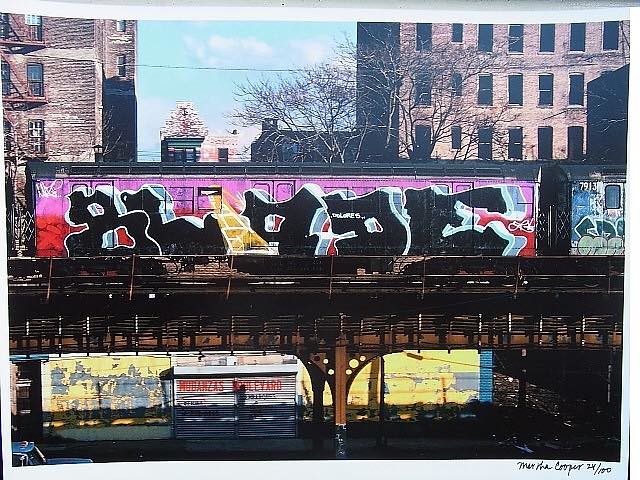The image is a color photograph in a landscape orientation, depicting an urban scene. It appears to be a photograph of a printed photograph, as evidenced by the white borders visible along the bottom, top, and slightly up the sides. In the bottom right corner of this white border is some illegible italic handwriting, possibly reading "May the Cooper" followed by "24/100," suggesting it might be an archival note or limited edition mark.

The focal point of the image is an elevated rail track with a rapid transit or subway car passing over it. The track's structure is composed of bronze or brown steel girders, reminiscent of Chicago's L train. The train car itself is prominently covered in graffiti, adorned with bubble-style black lettering outlined in white on a pink or purple background, stretching across its entire side. 

In the background, between the raised rail structure and the high-rises, a patch of sky is visible, light blue with soft white and grey clouds. There are barren trees with no leaves, suggesting the season could be late fall, winter, or early spring. On the left side of the image, a red brick high-rise building with a classic North American fire escape of bronze metal platforms and diagonal stairs is partially cut off at the top, while another high-rise occupies the right side.